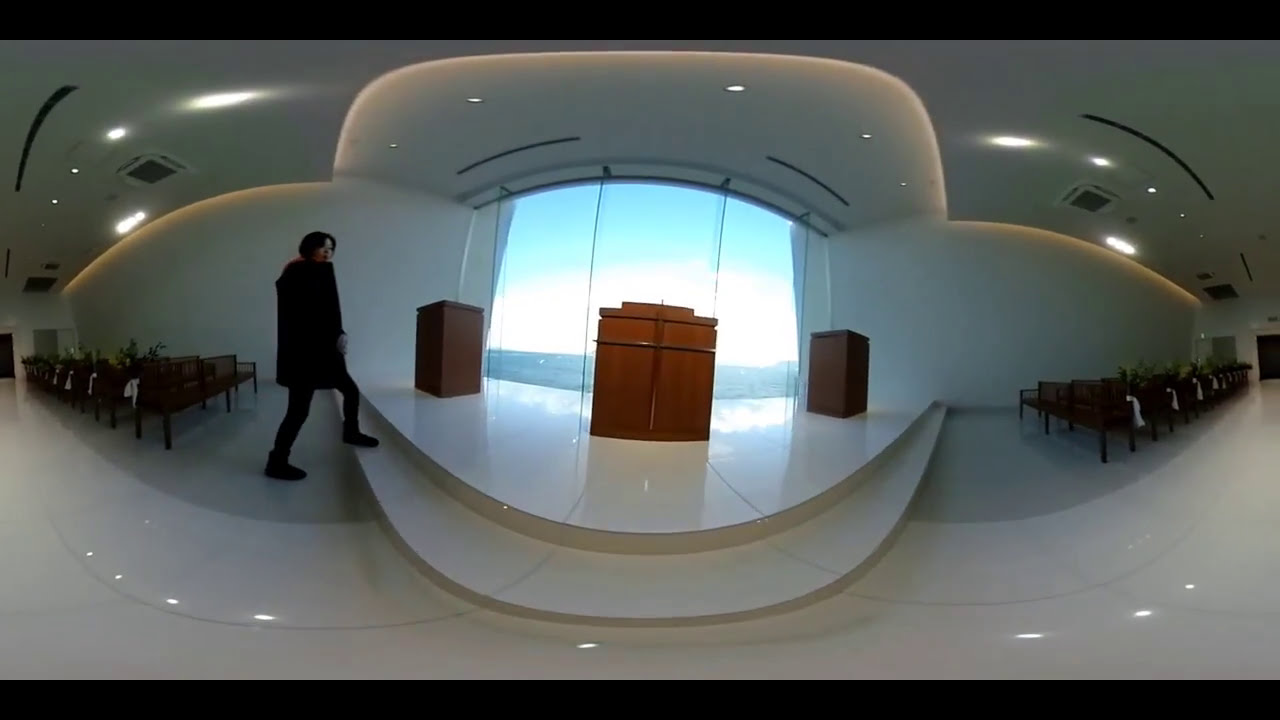In this image, we see the interior of a brightly lit, white-walled building with a glossy white floor, likely a church or conference room. The photograph, taken with a fisheye lens, captures a central stage flanked by benches or chairs, possibly made of wood in shades of black or brown, adorned with green leaves and white flowers at their ends. A person dressed in an all-black outfit is stepping up a two-stair stage, heading towards three wooden podiums of various shades of brown arrayed in the center. Behind these podiums is a large window, accentuated by a uniquely shaped wall, revealing an outdoor scene with a blue sky and darker regions where the landscape is visible. The symmetrical arrangement and absence of text contribute to the serene and formal atmosphere of the room.